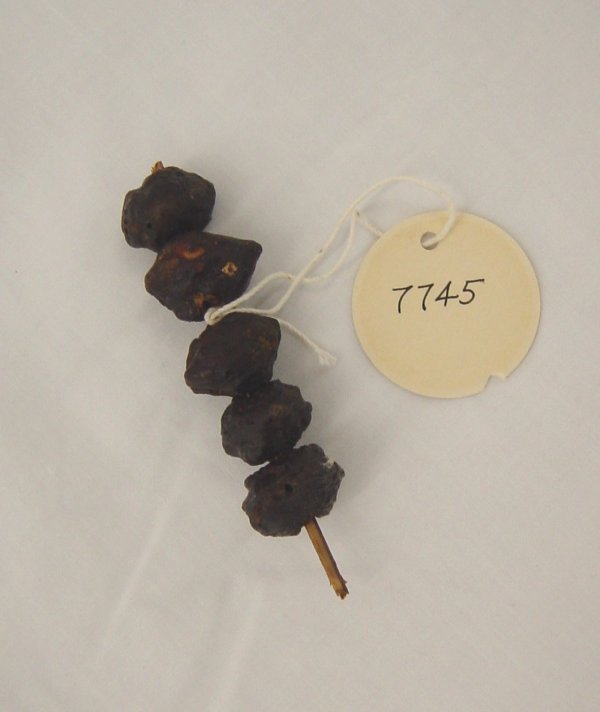The image appears to be a photograph of an art object, possibly part of a museum exhibit, indicated by a circular label bearing the number 7745. This label, likely for inventory purposes, is affixed to the object via a string. The object itself consists of what seem to be five weathered, rock-like elements, attached sequentially along a rough, twig-like stick. The rocks, or possibly other organic materials, exhibit a severely weathered appearance with dark, charred tones of brown and maroon. The string is tied between the second and third elements, displaying the tag which is slightly damaged at the bottom right corner. The entire arrangement is placed against a white, cloth-like surface, adding a clean backdrop to the rustic and worn aesthetic of the object.